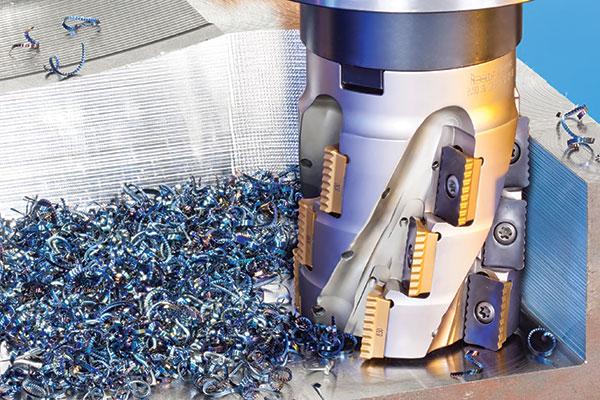This image depicts a large, complex mechanical device, predominantly situated on the right side of the photograph. The main component resembles a cylindrical drill bit with a solid silver top bordered by a dark gray baseline around 2 inches thick. This section leads into a barrel that features two contoured sections where it bulges out and retracts back in. The cylindrical drill bit is adorned with sets of three yellow, bristle-like devices, which appear to be screwed into the main component using six-sided Phillips head screws. There are three such sets – one on the far left, one in the middle, and one on the far right.

On the left side of the image, there is a substantial accumulation of metal shavings in a range of colors, including blues, purples, silvers, and whites. This splash of color contrasts with the metallic sheen of the device. The background includes a loom-like design and a wooden tabletop with additional scattered metal shavings, further emphasizing the industrial setting. Surrounding the complex drill bit and scattered shavings are various elements including blue, white, and gold-colored parts that add to the visual richness and complexity of the scene.